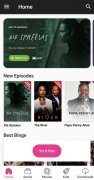The image appears to be a low-resolution, pixelated screenshot of a mobile website displayed in portrait mode. At the top, there's a black header containing the word "Home." To the left of this text are a few white lines, presumably representing a menu icon, and to the right is a white magnifying glass icon indicating a search function.

Below the header, there's a thumbnail section featuring a woman on the right side of the frame looking towards the left. The background of this thumbnail is green, and there is white text next to the woman, although it is difficult to decipher due to the low resolution. It seems to spell out something like "SIF SPREELASI." Directly beneath this text is a green button.

Further down, the section labeled "More Episodes" displays several additional small images or posters, each showing different individuals, likely promoting various shows. Below these posters, there's some black text that is challenging to read but seems to say "Best Binge."

At the bottom of the image, there's a purplish-pink button that appears to read "Try it Free." Finally, the bottom navigation bar contains five different icons. The first icon on the left, highlighted in purple, is labeled "Home." The remaining icons, with labels and symbols above them, represent other sections of the website.